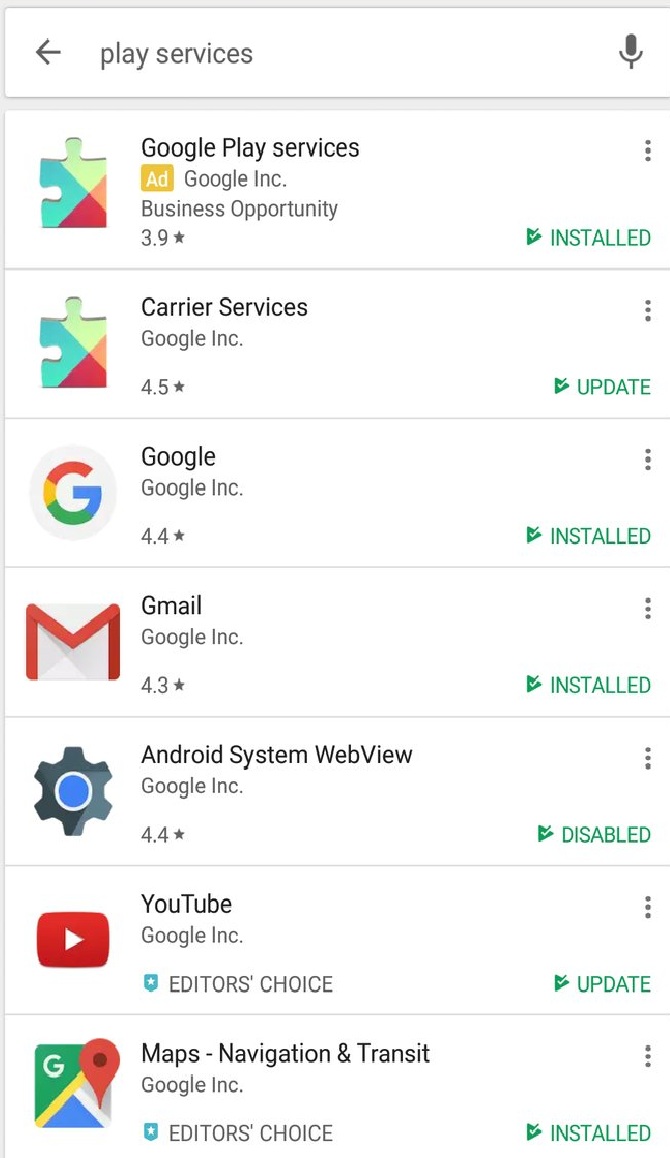Screenshot from an Android phone displaying the Google Play Store search results for "Play Services." At the top left, there’s a back arrow next to the phrase "Play Services." To the right, a microphone icon is visible. 

The list of search results includes:

1. **Google Play Services**  
   - **Logo:** Puzzle piece  
   - **Developer:** Google Inc.  
   - **Rating:** 3.9 stars  
   - **Status:** Installed  
   - **Type:** Ad  

2. **Carrier Services**  
   - **Logo:** Another puzzle piece  
   - **Developer:** Google Inc.  
   - **Rating:** 4.5 stars  
   - **Status:** Update available  

3. **Google**  
   - **Logo:** The iconic multicolored "G"  
   - **Developer:** Google Inc.  
   - **Rating:** 4.4 stars  
   - **Status:** Installed  

4. **Gmail**  
   - **Logo:** An envelope with a red "M"  
   - **Developer:** Google Inc.  
   - **Rating:** 4.3 stars  
   - **Status:** Installed  

5. **Android System WebView**  
   - **Logo:** A gear-like robot with a blue circle  
   - **Developer:** Google Inc.  
   - **Rating:** 4.4 stars  
   - **Status:** Disabled  

6. **YouTube**  
   - **Logo:** Red square with a white play button  
   - **Developer:** Google Inc.  
   - **Rating:** Editor's Choice  
   - **Status:** Update available  

7. **Google Maps - Navigation & Transit**  
   - **Logo:** A square, divided into segments: top and left are green with a "G," a yellow line, a blue bottom triangle, and a white right triangle featuring a red place marker  
   - **Developer:** Google Inc.  
   - **Rating:** Editor's Choice  
   - **Status:** Installed